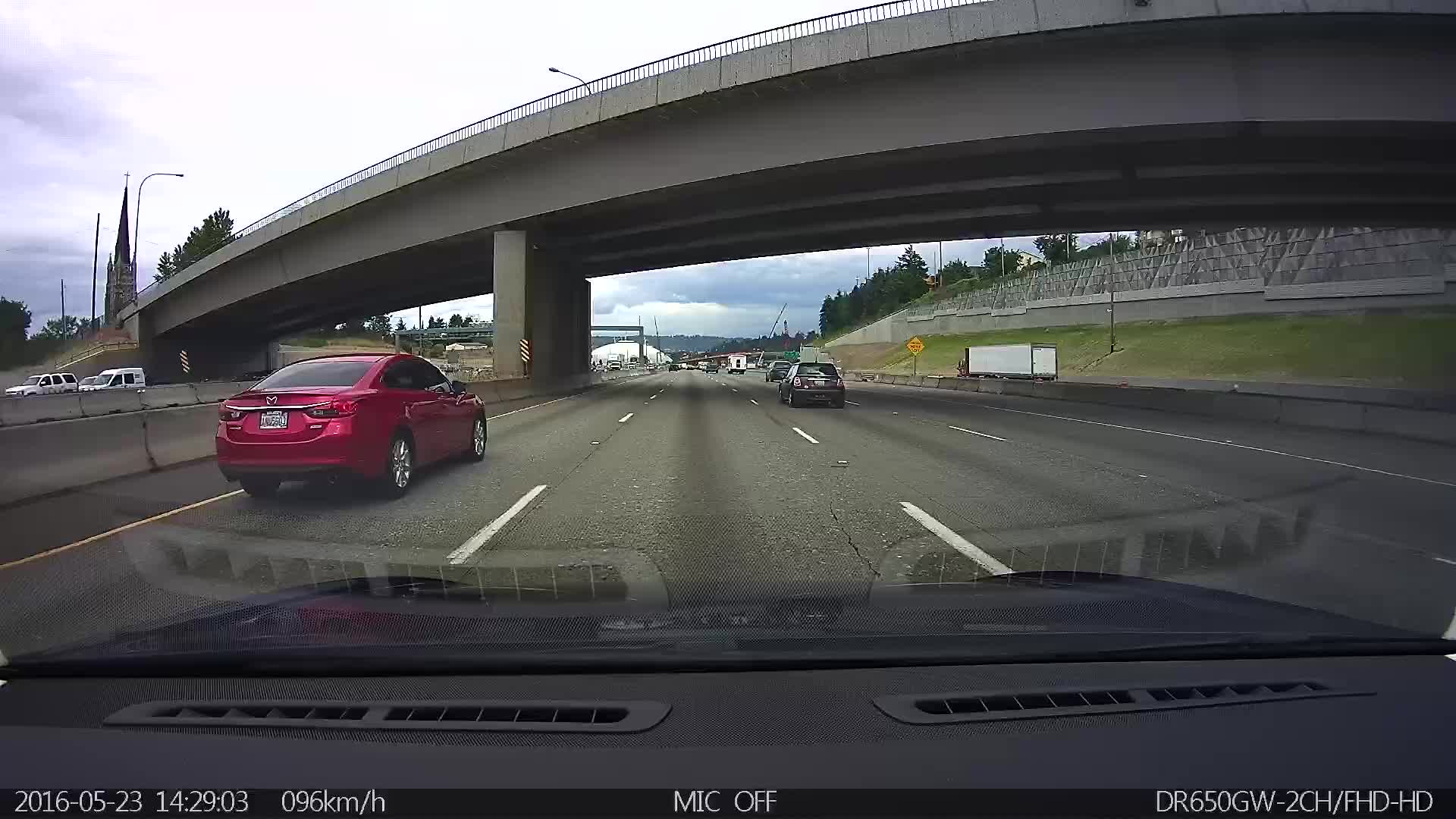In this high-resolution color photograph, likely captured by a dash cam, we observe the front view from a vehicle traveling on a four-lane highway. The image is stamped with the date "2016-05-23" and the time "14:29:03" at the bottom left corner, indicating the moment captured. The speed of the vehicle is displayed as 96 kilometers per hour, and the dash cam information reads "MIC OFF" and "DR650GW-2CH-FHD-HD" at the bottom right, suggesting the camera model. Central to the scene is an overpass bridge that the car is approaching. In the left lane next to the viewer’s vehicle is a red sedan, while further ahead in the right lane is a black vehicle. More vehicles are visible in the distance and on the other side of the highway. A concrete sound barrier wall lines the highway, behind which trees are visible. The distant skyline features a dome, potentially a sports arena, along with hills and trees. A church spire is noticeable on the left side, standing behind the overpass. This image, wider than it is tall, also captures the vehicle’s dashboard at the bottom edge, emphasizing the perspective from within the car.